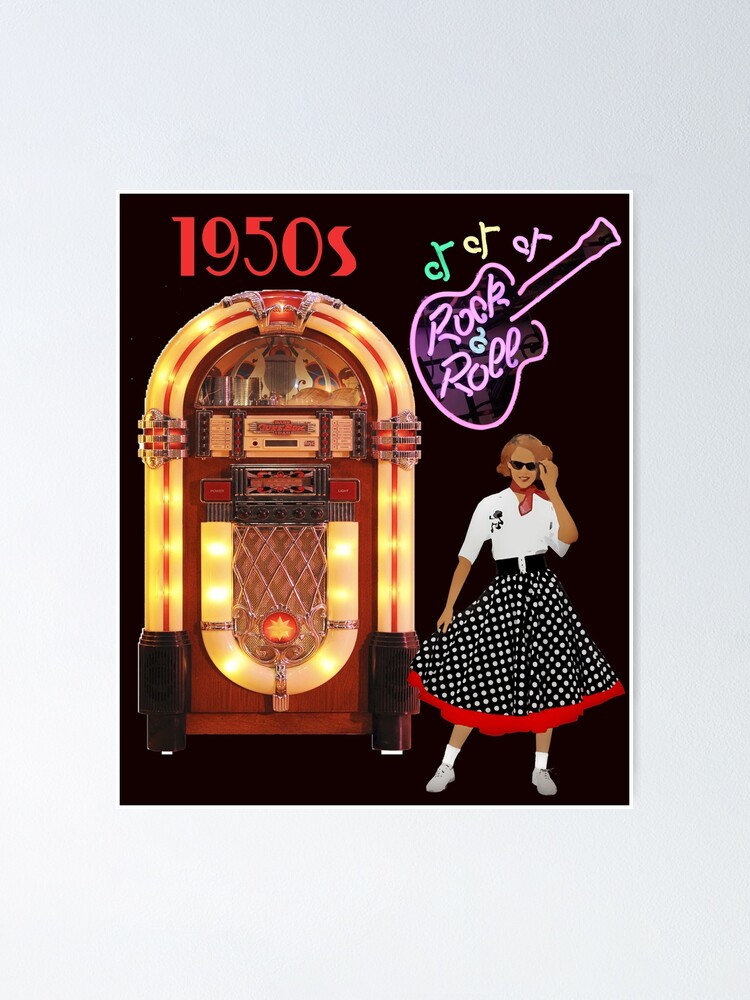The image depicts a vibrant, cartoon-style illustration set against a black background, reminiscent of a lively 1950s scene. On the left side, a large, illuminated jukebox with yellow-golden trim and a wooden face features a small window showcasing the records inside. It has a metal grating beneath a branded plate at the center. Above the jukebox, "1950s" is prominently displayed in bright red, stylized mid-20th-century font. On the right side of the image, a neon electric guitar shapes the words "rock and roll," with the guitar in pink and the text in vibrant green, accompanied by three colorful music notes in green, yellow, and purple. Below this neon display stands a young woman in a 1950s attire: she wears black sunglasses, a white top, a short red ascot, and a voluminous black-and-white polka dot skirt with a red hem. She completes her look with white socks and possible sneakers, embodying the lively spirit of the rock and roll era.